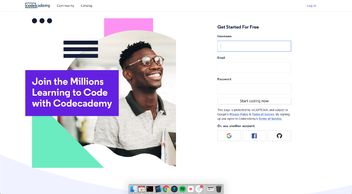This screenshot captures a promotional webpage from Code Academy, displaying a compact and difficult-to-read layout. In the top-left corner of the page, there's an indecipherable logo accompanied by two clickable words, both also unreadable. Central to the image is a photograph of a Black man with glasses, donning a gray shirt featuring a black stripe across the chest and a gray collar with buttons.

To the left of the man's photo, the text reads: "Join the Millions Learning to Code with Code Academy." On the right-hand side, a call-to-action message states: "Get Started for Free," above which three text boxes, though blurry and unreadable, are visible, likely intended for user input. Below these text boxes, a presumed submit button appears.

Further down, icons for authentication via Google and Facebook are visible, along with an unclear third option. At the very bottom of the screenshot, the computer's menu bar is partially visible, featuring recognizable icons for the calendar, Google Chrome, and YouTube, alongside several unidentified ones. Despite zooming in, the small size and blurriness of the text make it difficult to decipher additional details.